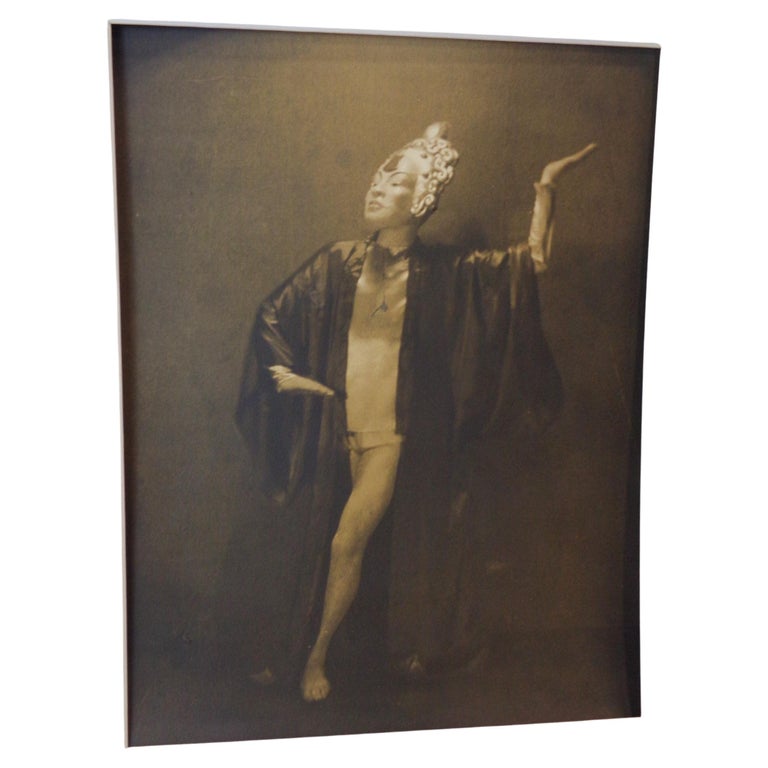This is an old, sepia-tinted black-and-white photograph of a performer, possibly engaged in a cultural dance. The individual appears to be female and is positioned against a background that shades from light gray in the center to darker gray towards the edges. She is dressed in an elaborate costume, featuring a curvaceous, metallic-looking headdress that loops around like fur hair or engraved golden locks. Her face is partially obscured by a shiny, intricate mask that adds an element of mystery.

The performer's attire includes a dark, silken robe draping elegantly to the floor and extending over her arms, complemented by numerous bracelets. Beneath the robe, she wears a very tight white shirt and very short shorts that resemble underwear, with one bare leg visible, crossing in front of the other. Her hands are artfully posed: one hand held up near her head with the palm turned upwards, and the other positioned by her waist with the palm facing down. This dramatic, dance-like pose, combined with her attire, suggests that she might be a dancer from a traditional cultural performance.